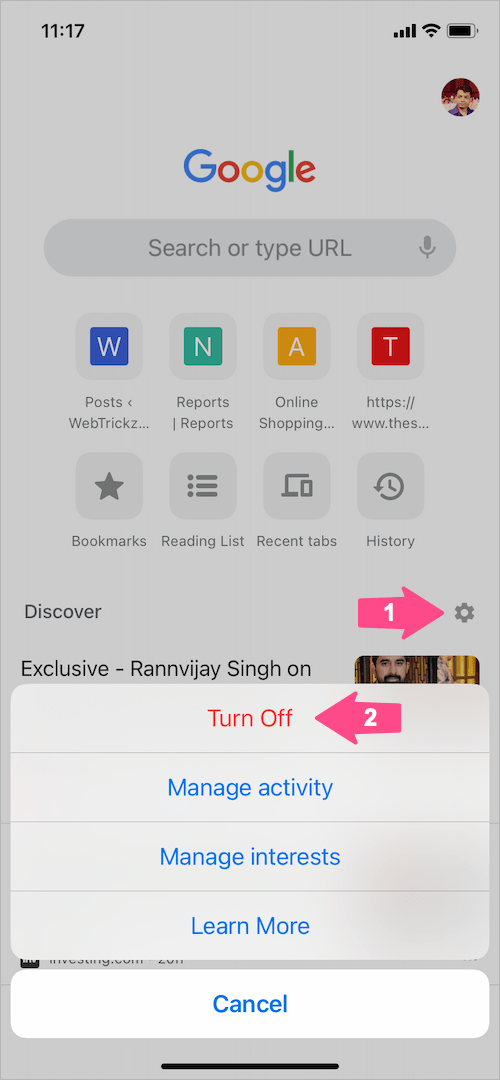The image is a screenshot from a smartphone, with the status bar displaying the date "11-17" at the top left corner and a nearly full battery icon. Beneath the status bar, there is a profile picture of a man. Centrally, the Google logo is prominently displayed above a gray search bar, which features a microphone icon on the right side. The text within the search bar reads "Search or type URL."

Below the search bar, there are various icons and labels: 

- To the left, a dark blue square with a white "W" inside it, labeled "Posts and Web Tricks."
- Next to it, a turquoise square with a white "N," labeled "Reports Reports."
- Adjacent to that, an orange square with a white "A," labeled "Online Shopping."
- Further right, a red square with a white "T" above a partially visible URL beginning with "https://www.thes..."

At the bottom of the screen, four icons are arranged horizontally. The first icon is a bookmark with a star symbol on the left side.